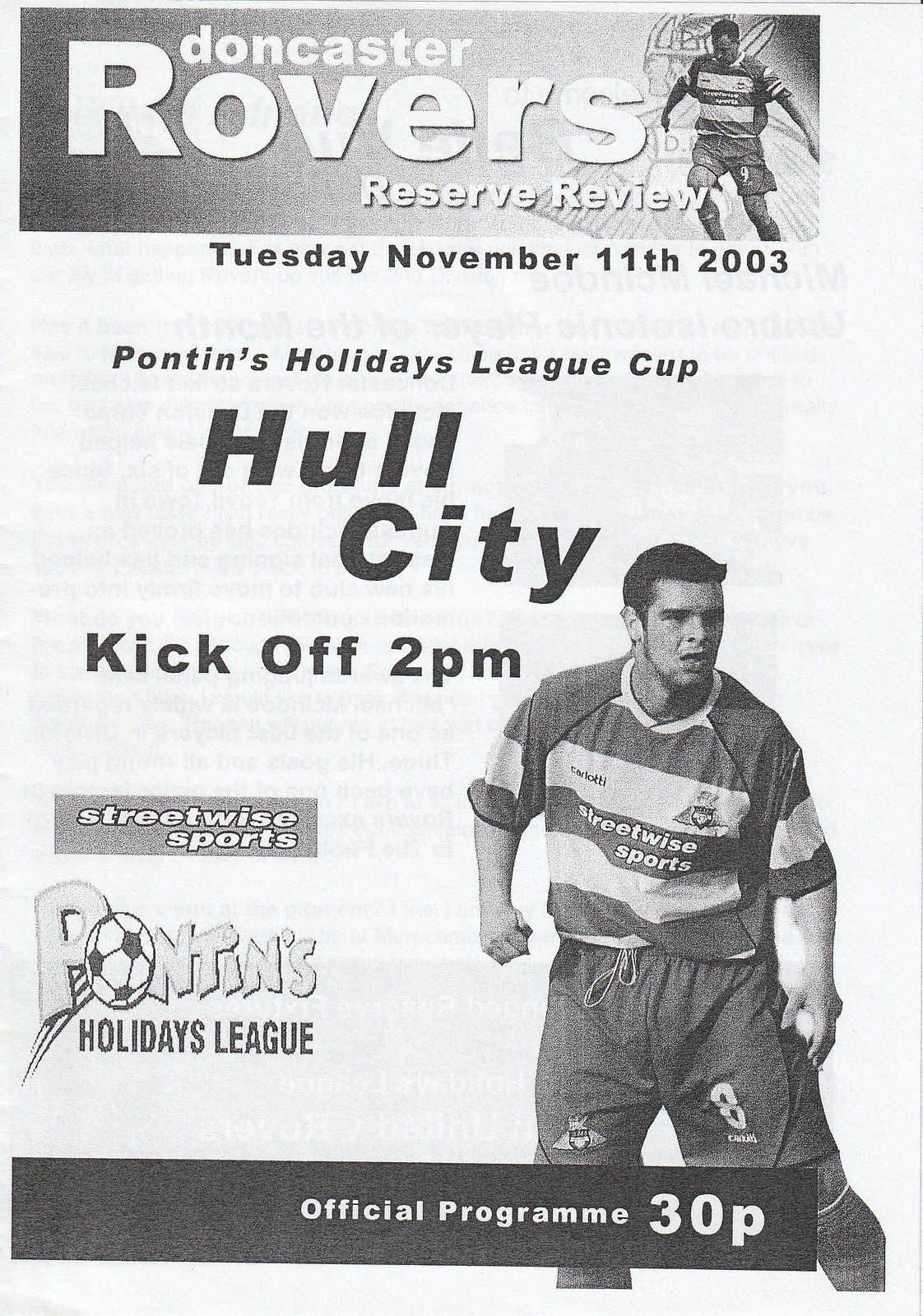This black and white program cover for a soccer match prominently features the banner "Doncaster Rovers Reserve Review" at the top. Below it, the date "Tuesday, November 11, 2003," is displayed, followed by "Pontins Holiday League Cup" and "Hull City." The kickoff time is listed as 2 p.m. On the lower right side, there's an image of a soccer player wearing a striped jersey with the number eight, high socks, and shorts, seemingly engaged in a match. In the left corner, a banner reads "Streetwise Sports," under which "Pontins Holiday League" appears with a soccer ball as the 'O.' At the bottom of the page, a banner indicates "Official Program 30P." The overall design resembles a monochromatic newspaper print.